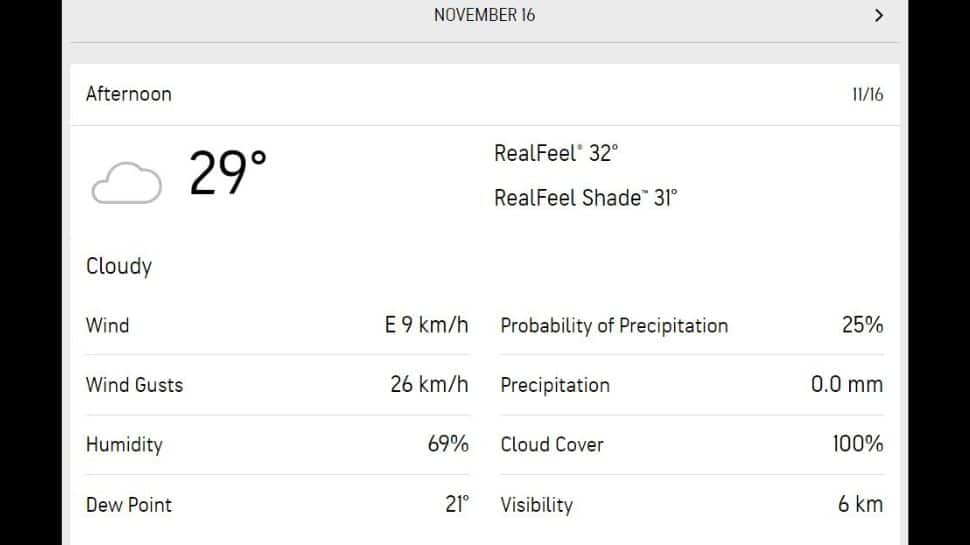The screenshot depicts a section of a weather-focused website with a meticulously organized layout. 

On both the left and right sides of the image, black vertical banners extend downward from the top edge. A horizontal grey banner spans the full width at the top, seamlessly intersecting with the black side banners. Centered within this grey banner, bold black text announces the date: "NOVEMBER 16" with "NOVEMBER" prominently in all capital letters. To the right of the date, a right-pointing arrow directs attention downward.

Beneath the grey banner, the background transitions to white. The word "Afternoon" is displayed in black text with a capitalized "A." Below this, the date "11/16" is clearly indicated.

Continuing downward, a horizontal line separates the date from weather details. Directly below the line, an icon of a cloud is shown with temperature data: "29 Degrees." Additional information includes "Real Feel: 32 Degrees" and "Real Feel Shade: 31 Degrees."

On the right side, more detailed weather data is presented: 
- "Cloudy" status
- Wind conditions: "Wind: E, 9 km/h" and "Wind Gust: 26 km/h"
- Humidity: 69%
- Dew Point: 21 Degrees
- Probability of Precipitation: 25%
- Precipitation: 0.0 mm
- Cloud Cover: 100%
- Visibility: 6 km

Each section of text begins with a capital letter for the words, except for the word "up," enhancing readability and emphasizing key weather statistics. The overall layout ensures that all relevant weather information is readily accessible and clearly organized for the user.